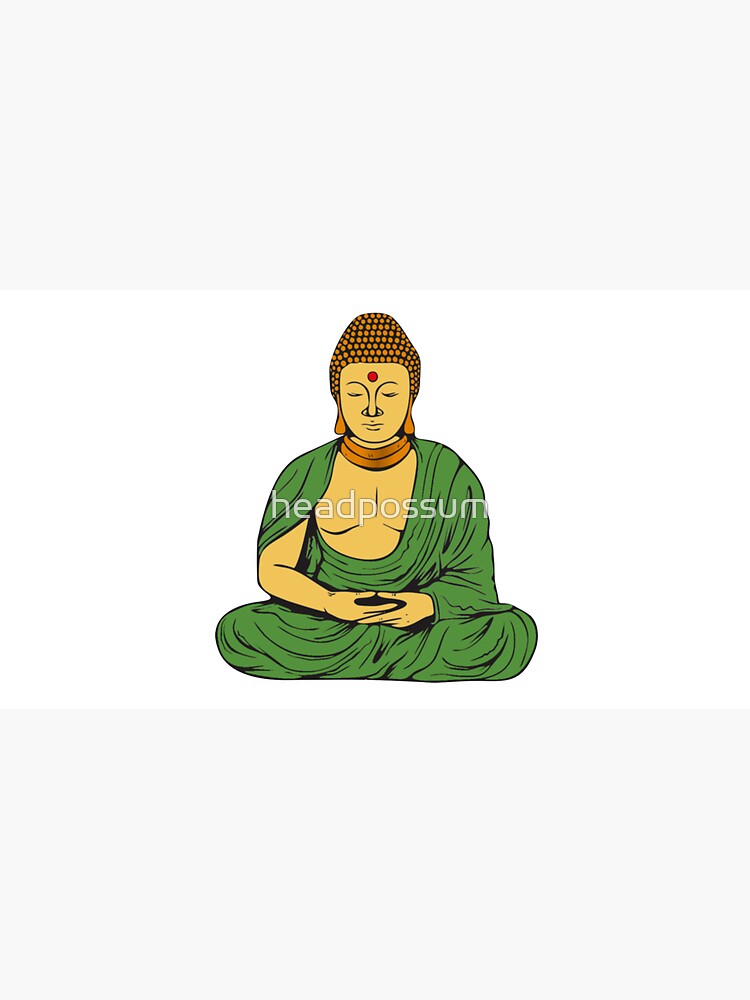The image depicts a serene, meditative figure against an entirely white background. The figure, potentially a Buddha-like man or female figure, is seated in an Indian-style pose, clad in a flowing green robe that drapes over their body, detailed with black lines that illustrate the robe's wrinkles. Around their neck, they wear two gold necklaces. The figure also has gold earrings and a complex headdress adorned with beaded jewelry, forming a pyramid-like structure without a point at the top. Their eyes are closed in deep contemplation, with a red bindi marking the center of their forehead. The background consists of three rectangles—a light reddish gray rectangle at the top and bottom, with a large white rectangle in the middle, framing the meditative figure centrally.